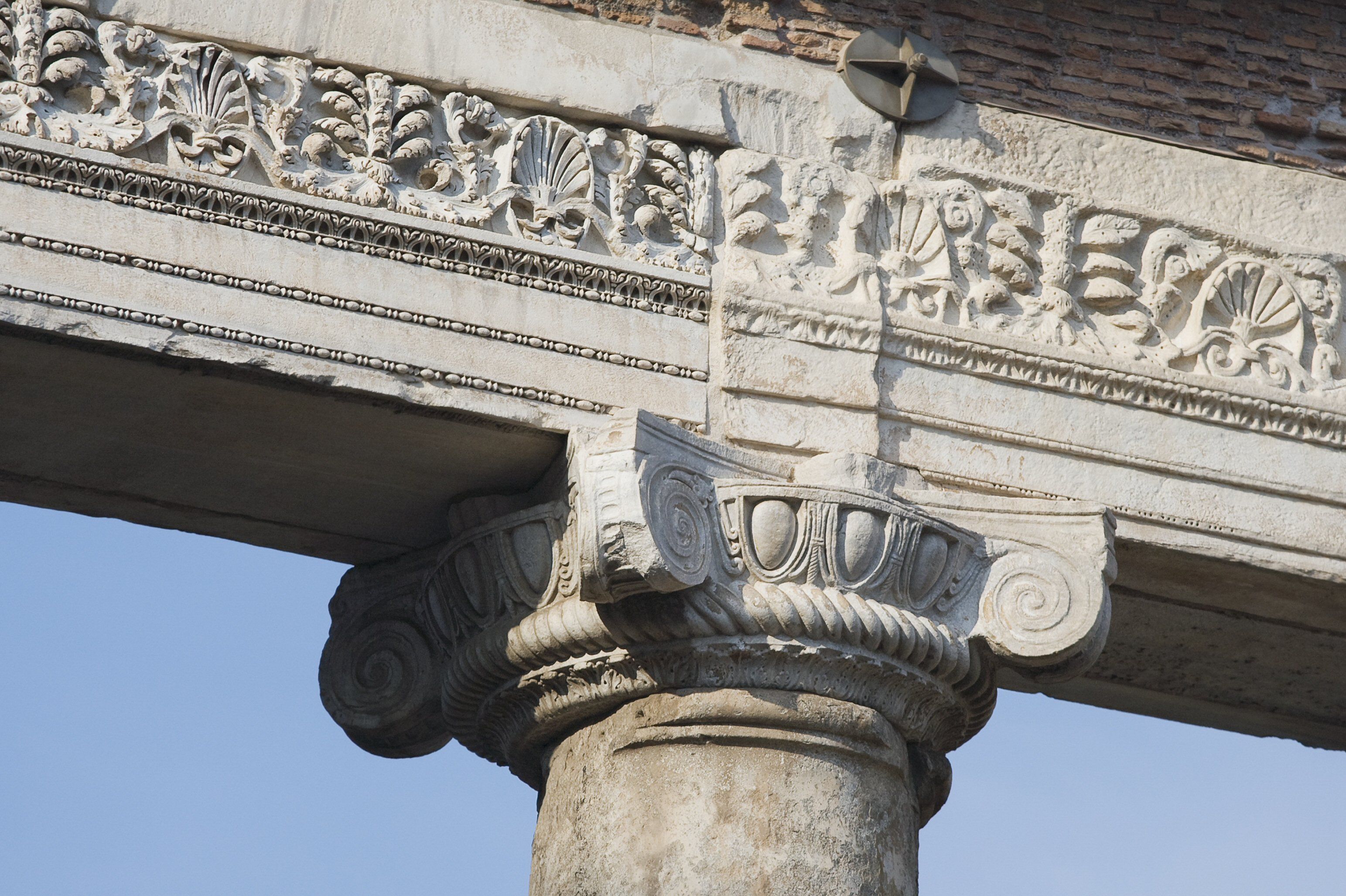This photograph captures the top portion of a large, ornate stone pillar supporting a lighter gray cement beam within an ancient or ruined structure. The pillar, exhibiting an older gray ceramic or concrete appearance, features intricate carvings, including ovals and swirling designs on either side. The top of the pillar rounds out into a circle, merging seamlessly with a highly detailed beam adorned with architectural symbols such as seashell motifs and leaf engravings. Above the beam, the structure transitions into a brick layer, where a metal circle with a cross design affixes the brick to the stone. The outdoor setting is evident by the clear blue sky in the background and the sunlight casting shadows on the left side, indicating the Sun is shining from the right.